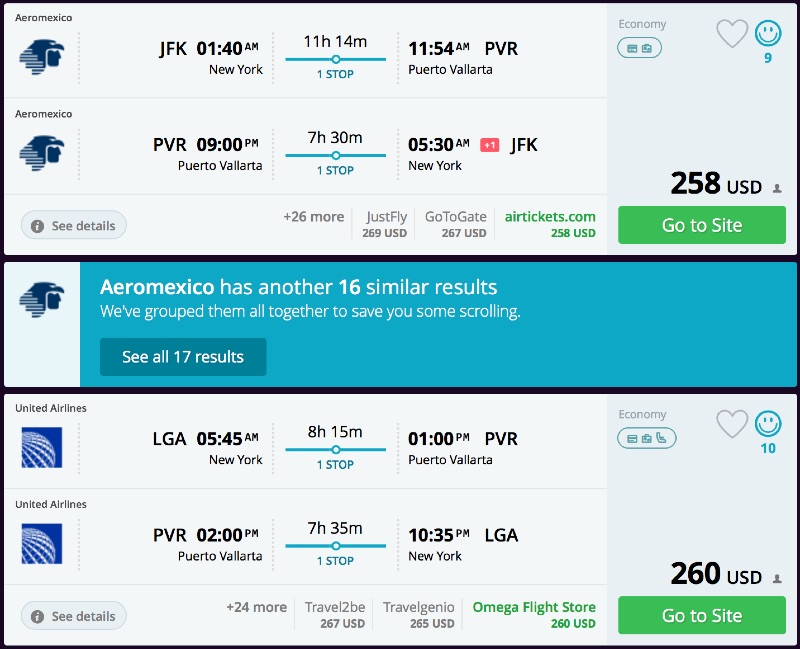The image appears to be a screen capture or a picture taken from a leaflet or brochure, showing flight schedule information, heavily outlined in black. The layout comprises three horizontal bars: two wide off-white bars at the top and bottom, and a narrower blue bar in the center.

### Top Section:
In the top off-white section, on the left, details for Aero-Mexico flights are presented:
- **Departing Flight:**
  - **Route:** JFK (New York) to PVR (Puerto Vallarta)
  - **Details:** One stop, highlighted in blue
- **Returning Flight:**
  - **Route:** PVR (Puerto Vallarta) to JFK (New York)
  - **Details:** One stop, highlighted in blue
- **Additional Info:** States "26 more" flight options available

The price options are listed as:
- "Just Fly" for $269
- "Go to Gate" for $267
- "Airtickets.com" for $258 (highlighted in green as the cheapest fare).

On the right side, the cheapest price ($258) is displayed in bold, accompanied by a green button with white lettering that says "Go to Site."

### Center Section:
In the central blue bar, a note says: "See all 17 results." This section mentions that Aero-Mexico offers another 16 similar results, grouped together to save scrolling.

### Bottom Section:
In the bottom off-white section, information for United Airlines flights is shown:
- **Departing Flight:**
  - **Route:** JFK (New York) to PVR (Puerto Vallarta)
  - **Details:** One stop
- **Returning Flight:**
  - **Route:** PVR (Puerto Vallarta) to JFK (New York)
  - **Details:** One stop
- **Additional Info:** States "24 more" flight options available

The price options are listed as:
- "Travel to B" for $267
- "Travel Genio" for $265
- "Omega Flight Store" for $260 (highlighted in green as the lowest fare).

On the right side, the cheapest price ($260) is displayed in bold, with a green "Go to Site" button in white lettering.

This detailed caption thoroughly describes the layout and content of the flight schedule information, emphasizing the available airlines, flight details, and pricing options, along with navigational aids and highlighted cost-efficient choices.